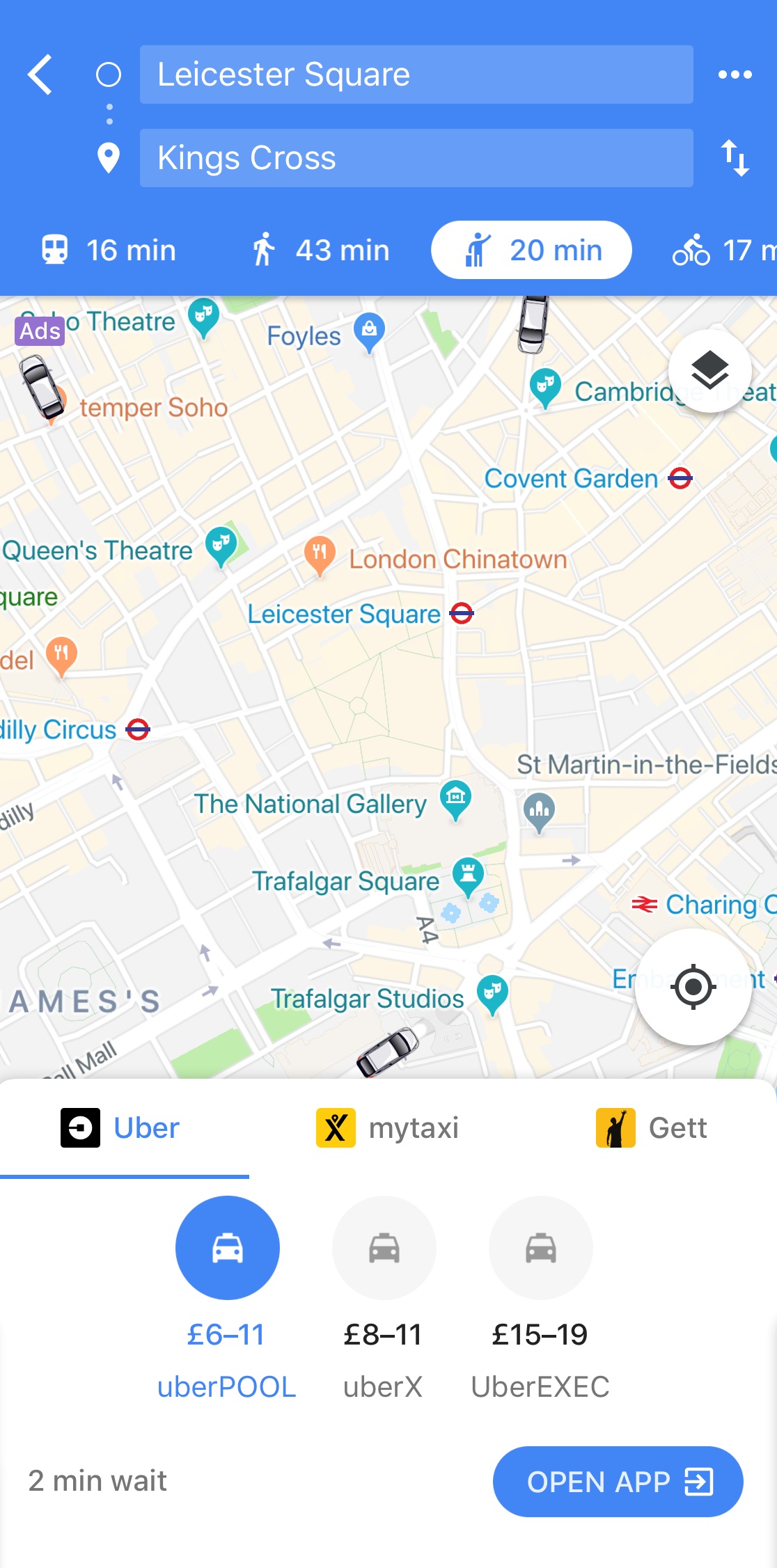This screenshot displays a map focused on a route from Leicester Square to King's Cross. At the top, there is a blue rectangle featuring a white arrow pointing left for navigating back. The map shows multiple transportation options and their respective travel times: 16 minutes by bus, 43 minutes walking, 20 minutes by cab, and 17 minutes by bike. 

In the upper left corner, the word "ads" is written in blue. The map highlights key landmarks such as Trafalgar Studios, Trafalgar Square, and the National Gallery, indicating the route involves heading straight up and then diagonally downward.

Below the map, transportation services like Uber, My Taxi, and GET are listed, showing fare estimates: £6-11 for UberPool, £8-11 for UberX, and £15-19 for UberExec, along with a 2-minute wait time and a prompt to open the app.